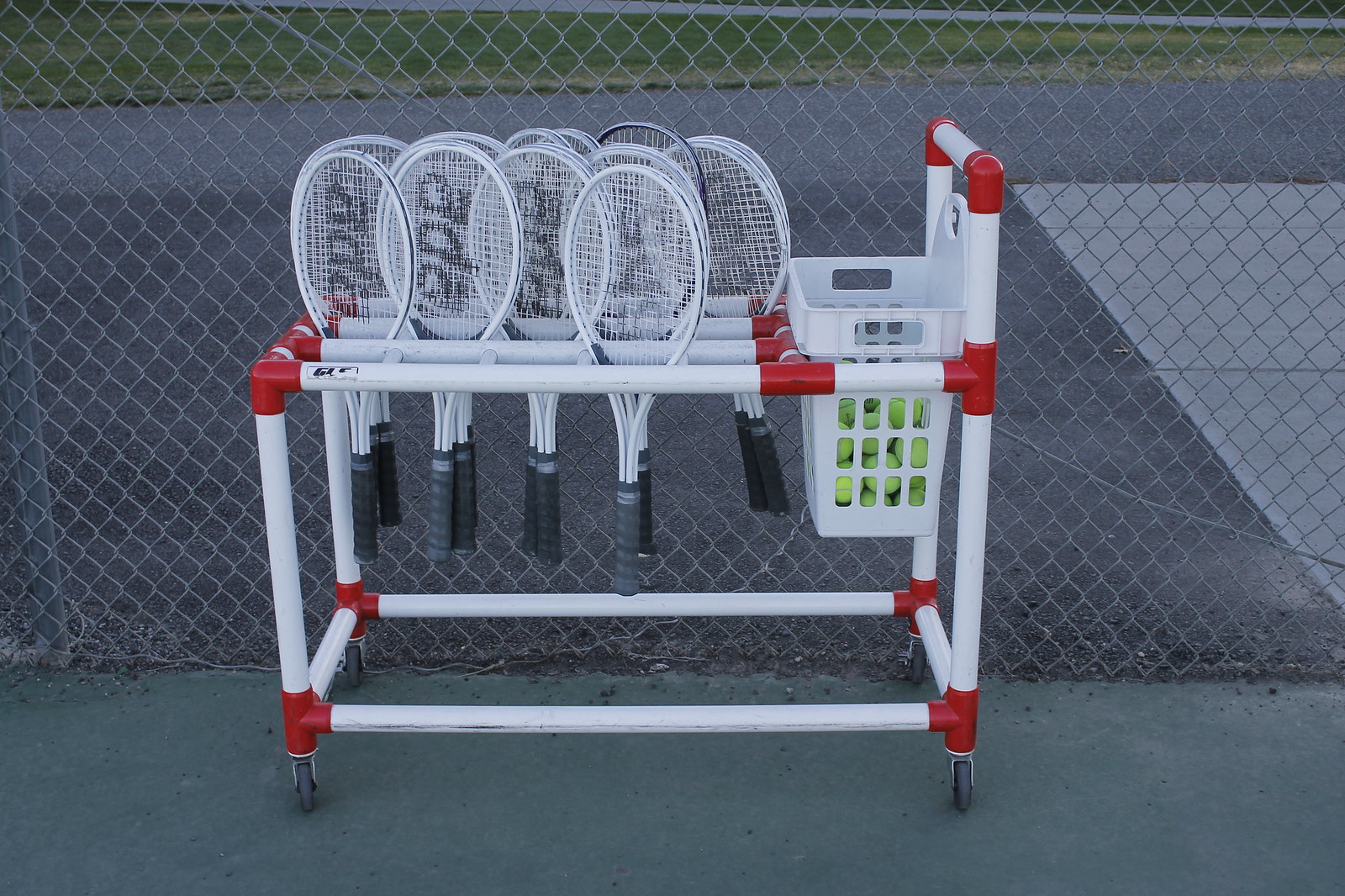The image depicts an outdoor tennis court with a green surface, bordered by a typical gray chain-link fence. On the court, there's a storage cart primarily constructed from white PVC piping, reinforced with red couplers at the corners and joints. This cart, designed for storing tennis equipment, has approximately 15 white tennis rackets, all featuring black handles and distinctive lettering in the netting. Adjacent to the rackets, on the right side of the cart, is a drop-down basket filled with traditional yellow-green tennis balls. The cart sits on four wheels and is positioned close to the fence, which separates the court from a concrete pavement and a strip of green grass visible in the background.